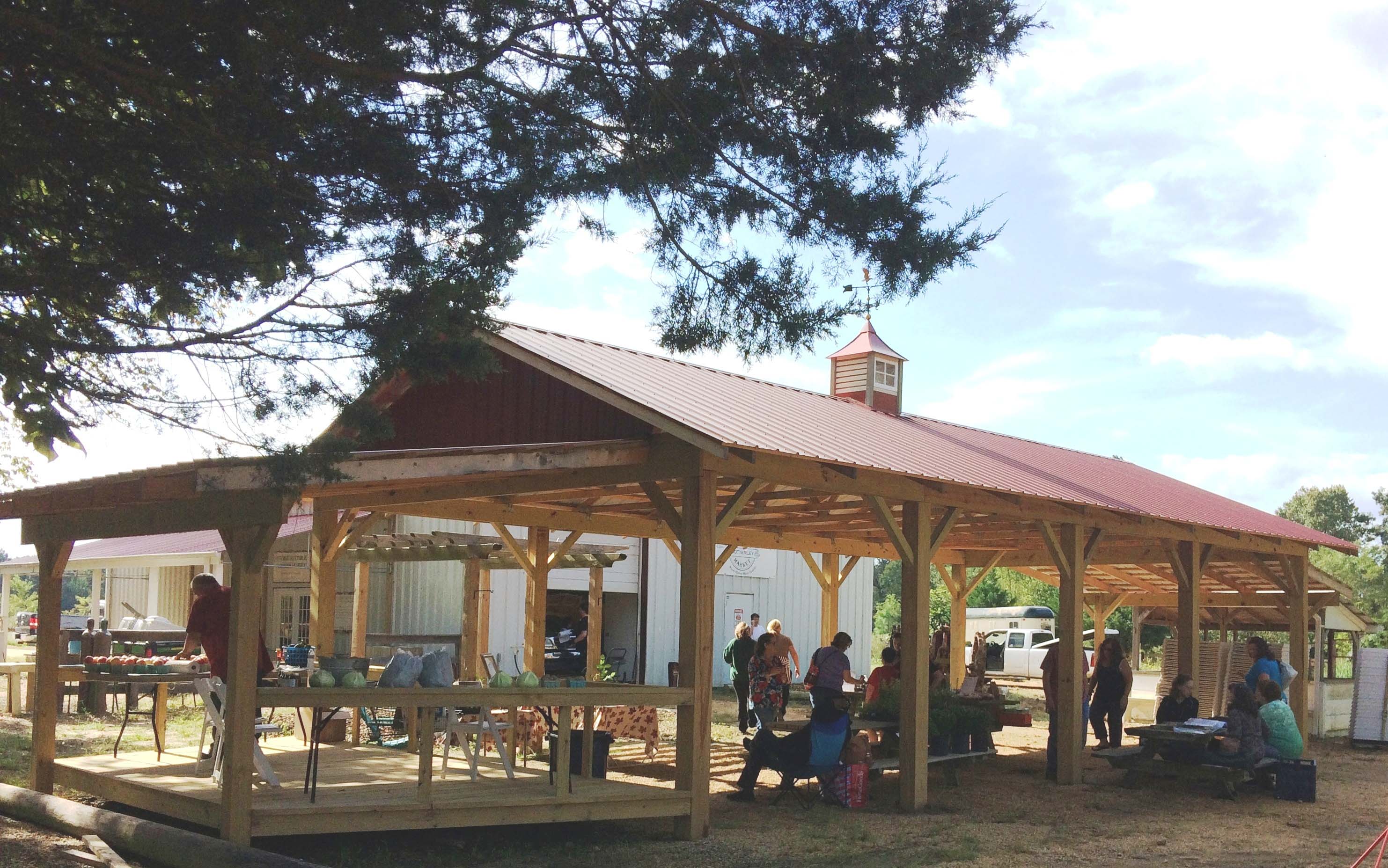In this rectangular photograph, we observe an outdoor scene likely set beneath a partially built barn or an open-air structure with a red roof supported by natural wooden beams. The setting appears to host a gathering or a small event, possibly an early stage of an outdoor market. Various chairs and two or three picnic tables are arranged within the space. 

To the left, a man stands in front of a table laden with baskets of what appear to be fruits or vegetables, suggesting the presence of vendors. Beyond this foreground structure, a one-story silver barn-like building with multiple doorways, including a double door, stands prominently, hinting at its use as part of the market or another functional space.

Approximately 12 to 13 individuals are scattered throughout the scene, either roaming, seated, standing, or engaged in conversation, emphasizing the communal and informal atmosphere. The warm weather is evident from the attire of several attendees dressed in short sleeves or tank tops. The backdrop reveals a lush expanse of green trees to the right, adding a picturesque natural element to the lively gathering.